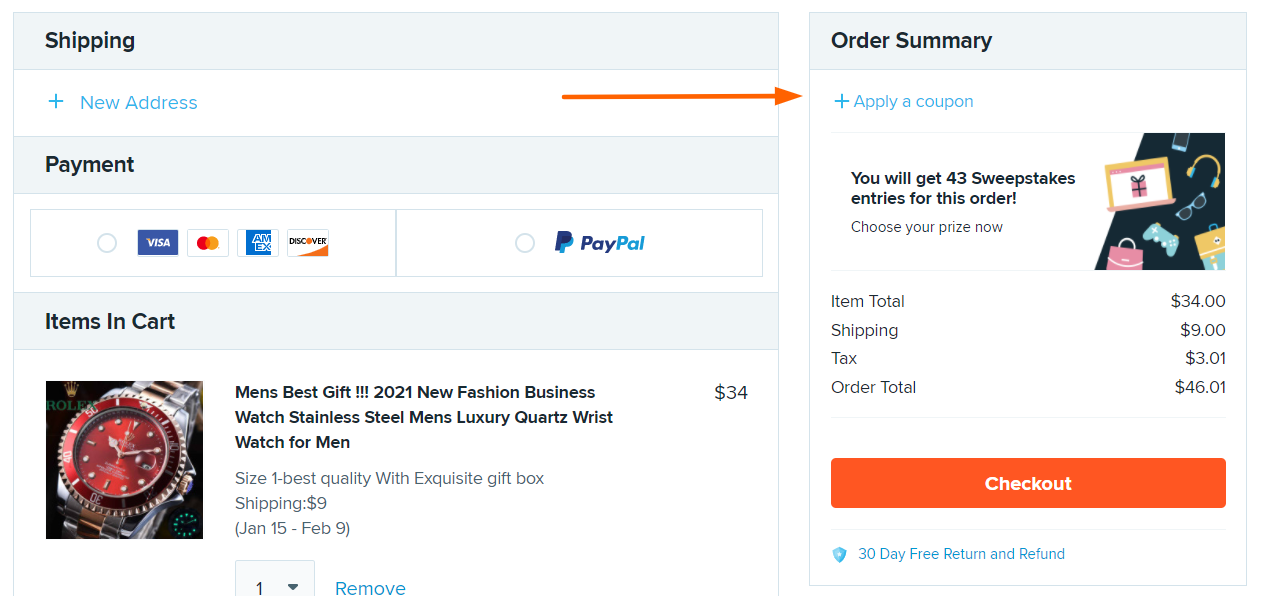The image depicts a checkout page of an e-commerce website, divided into two main sections. On the left, there is a shipping field with various options for the user to select. On the right, there is an order summary, highlighted by an orange arrow overlay pointing towards it.

Starting with the order summary, at the top, there's a blue-text link featuring a plus sign labeled "Apply a Coupon." Below this, an advertisement mentions that the user will receive 43 sweepstake entries for this order and prompts them to choose their prize now, with graphical icons representing purses, video games, and sunglasses to the right.

Following the advertisement are four lines detailing the cost breakdown for the order:
- Item Total: $34
- Shipping: $9
- Tax: $3.01
- Order Total: $46.01

Below the cost breakdown, there is an orange, wide horizontal checkout button with white text that reads “Checkout." Underneath this button, there's a note stating "30 days free return or refund."

On the left side, under the shipping field, the order section starts with an input for a new address followed by payment options. It features a selection circle where users can choose from Visa, MasterCard, American Express, and Discover Card logos. To the right of these options, there is an additional option for PayPal.

Further down, the details of the item in the cart are displayed:
- Item: Men's Best Gift
- Year: 2021
- Description: New Fashion Business Watch, Stainless Steel Men's Luxury Quartz Wristwatch for Men, Size: One, Best Quality with Exquisite Gift Box
- Price: $34
- Shipping: $9
- Estimated Delivery: January 15th to February 9th
- Image: A watch with a red face

This comprehensive layout guides the user efficiently through the checkout process while providing a detailed summary of their order.